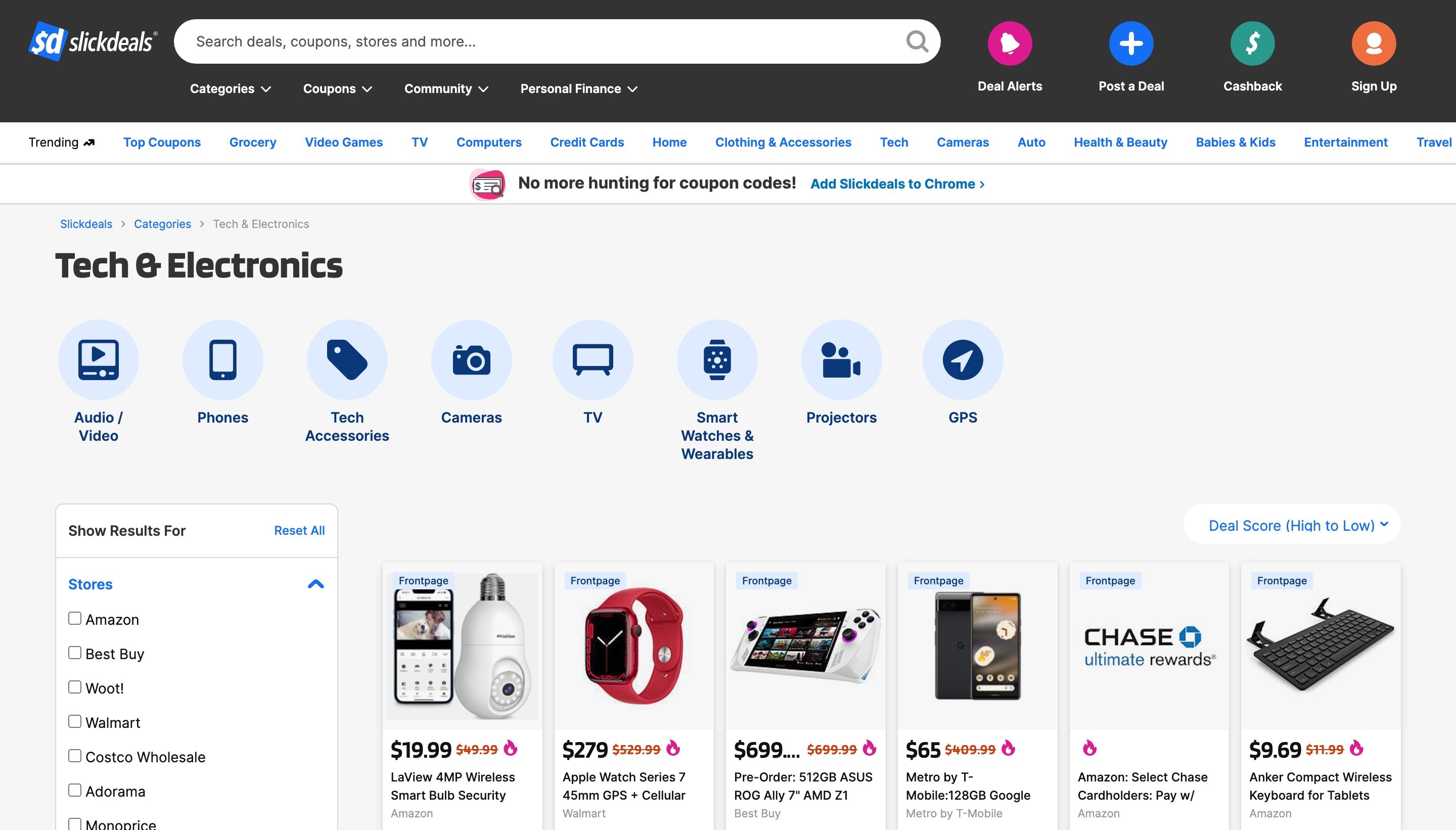This image showcases the homepage of the Slick Deals website. At the very top, a prominent horizontal black bar stretches across the screen, emblazoned with the Slick Deals logo. To the right of the logo, there is a search bar, and next to it, four distinct buttons in varying colors: a pink "Deal Alerts," a blue "Post a Deal," a green "Cash Back," and an orange "Sign Up." 

Below this navigation bar, the site offers a wide array of categories for users to explore, listed in blue text: Top Coupons, Grocery, Video Games, TV, Computers, Credit Cards, Home, Clothing, Accessories, Tech, Cameras, Auto, Health and Beauty, Babies and Kids, Entertainment, and Travel. The focus shifts to tech and electronics, displaying icons representing various subcategories such as Audio and Video, Phones, Tech Accessories, Cameras, TVs, Smart Watches and Wearables, Projectors, and GPS devices.

Following these categories, there is a visually engaging row of six promotional images. The first image features a wireless smart bulb, followed by an Apple Watch. The third image displays a handheld computer game, while the fourth shows a cell phone. The fifth image appears to be an advertisement for Chase Ultimate Rewards, and the sixth showcases a compact wireless keyboard designed for tablets. This layout provides users with an overview of current popular deals and advertisements on the Slick Deals website.